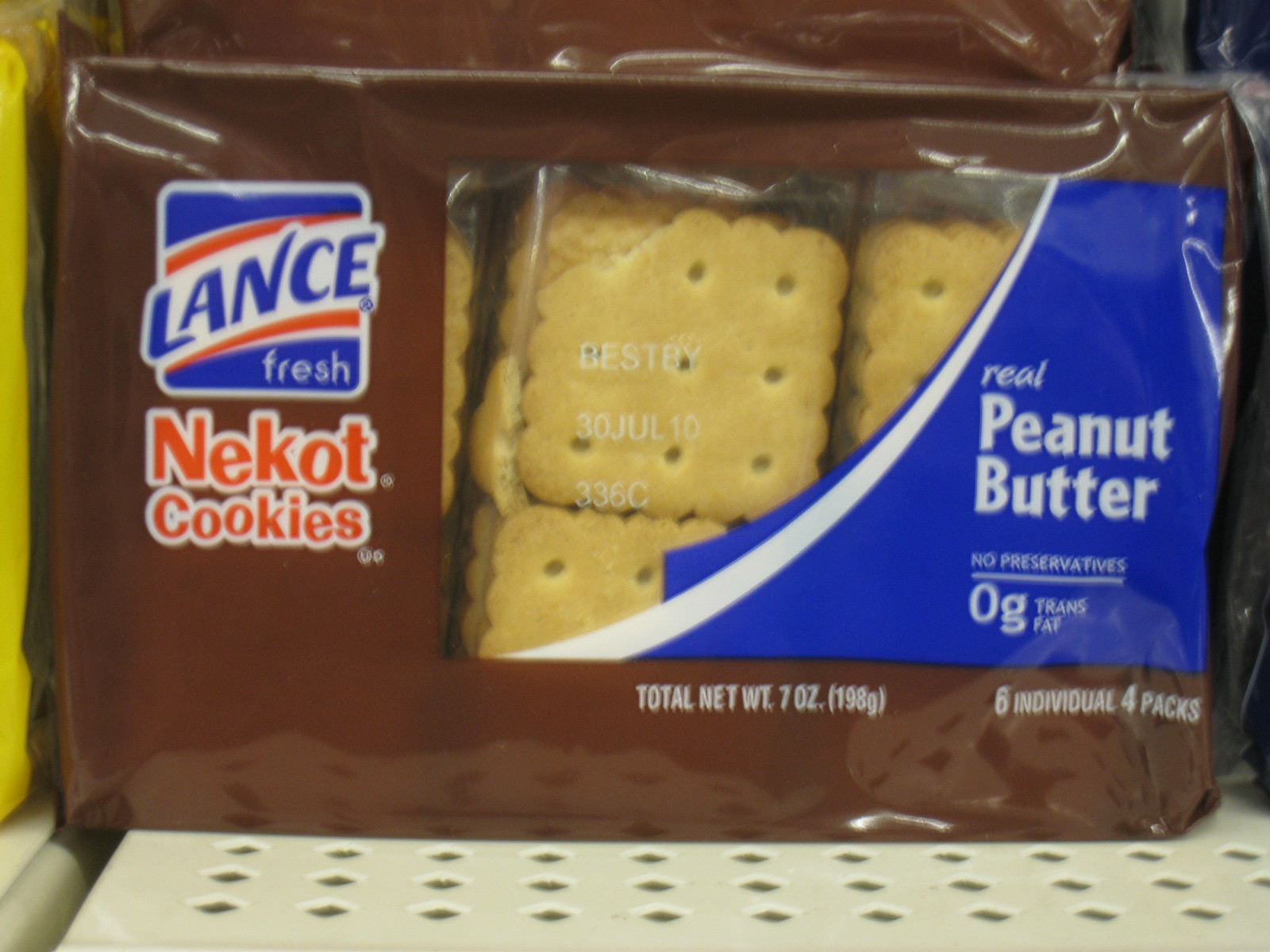The image features a package of Lance Fresh Nekot Cookies, prominently displaying its high-quality ingredients: real peanut butter, no preservatives, and zero grams of trans fat. The brown packaging includes the Lance Fresh logo, which is designed in blue with horizontal white and red streaks. A transparent cutout at the center of the packaging offers a tantalizing glimpse of the cookies inside. The "Best By" date, printed as "Best By 30 JUL," indicates that the cookies are best consumed by July 30th, 2010. In the bottom right corner, it is noted that the package contains six individual packs, each with four cookies.